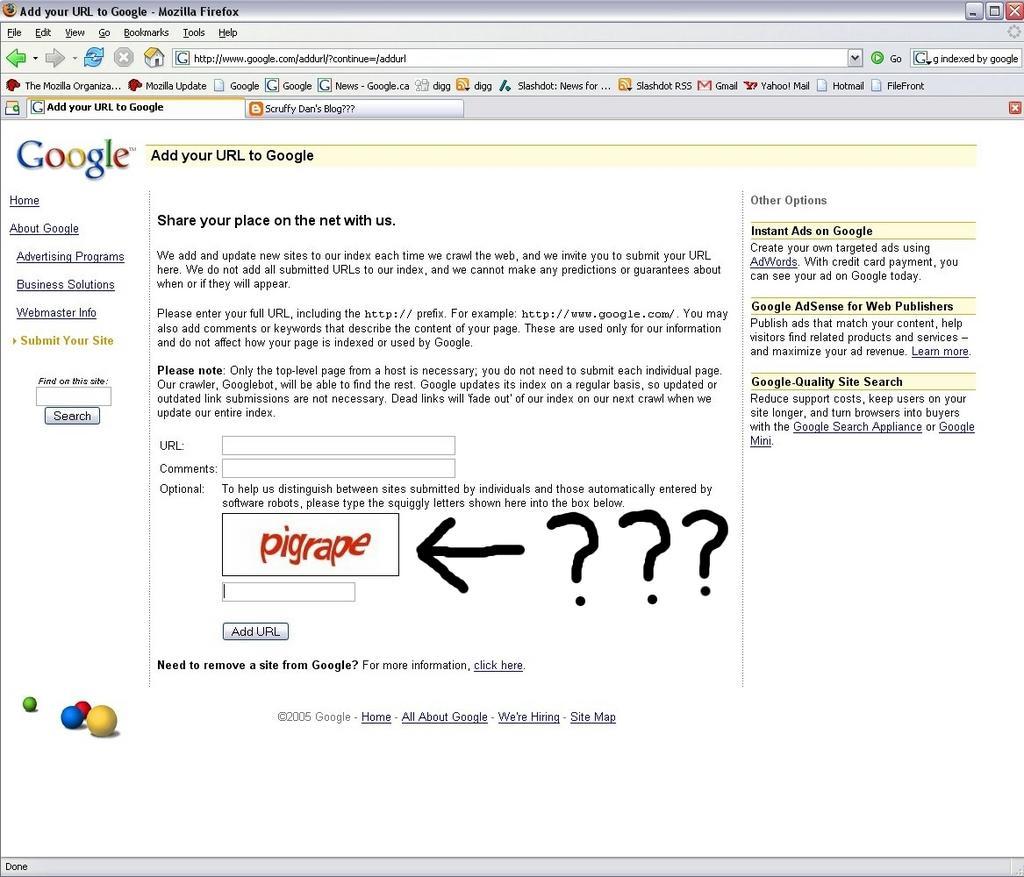The image is a color screenshot taken from a website, displaying a web form for adding a URL to Google using Mozilla Firefox. At the top of the browser window, the title "Add Your URL to Google" is prominently displayed. In the right-hand corner, there are minimized and exit buttons, along with a maximize button.

The browser's menu bar is visible and includes options such as File, Edit, View, Go, Tools, and Help. Below this, the toolbar features forward and back buttons, a refresh button, a next button, and a home button.

The main content of the webpage shows Google’s URL submission form. The headline reads "Add your URL to Google – Share your place on the net with us." Below this headline, various text blocks are present, though their content is illegible due to small print.

The form includes a field labeled "Enter your URL" along with an optional comments section. Additionally, there is a CAPTCHA security feature displayed in red text, with the phrase "PI GRAPE" (P I G R A P E). Beside the CAPTCHA, a black arrow points towards it, accompanied by three black question marks.

At the bottom of the form, there is a checkbox labeled "Never," along with a button that says "Add URL." There is also a link offering the option to "Remove from Google," indicating users can click here for removal instructions.